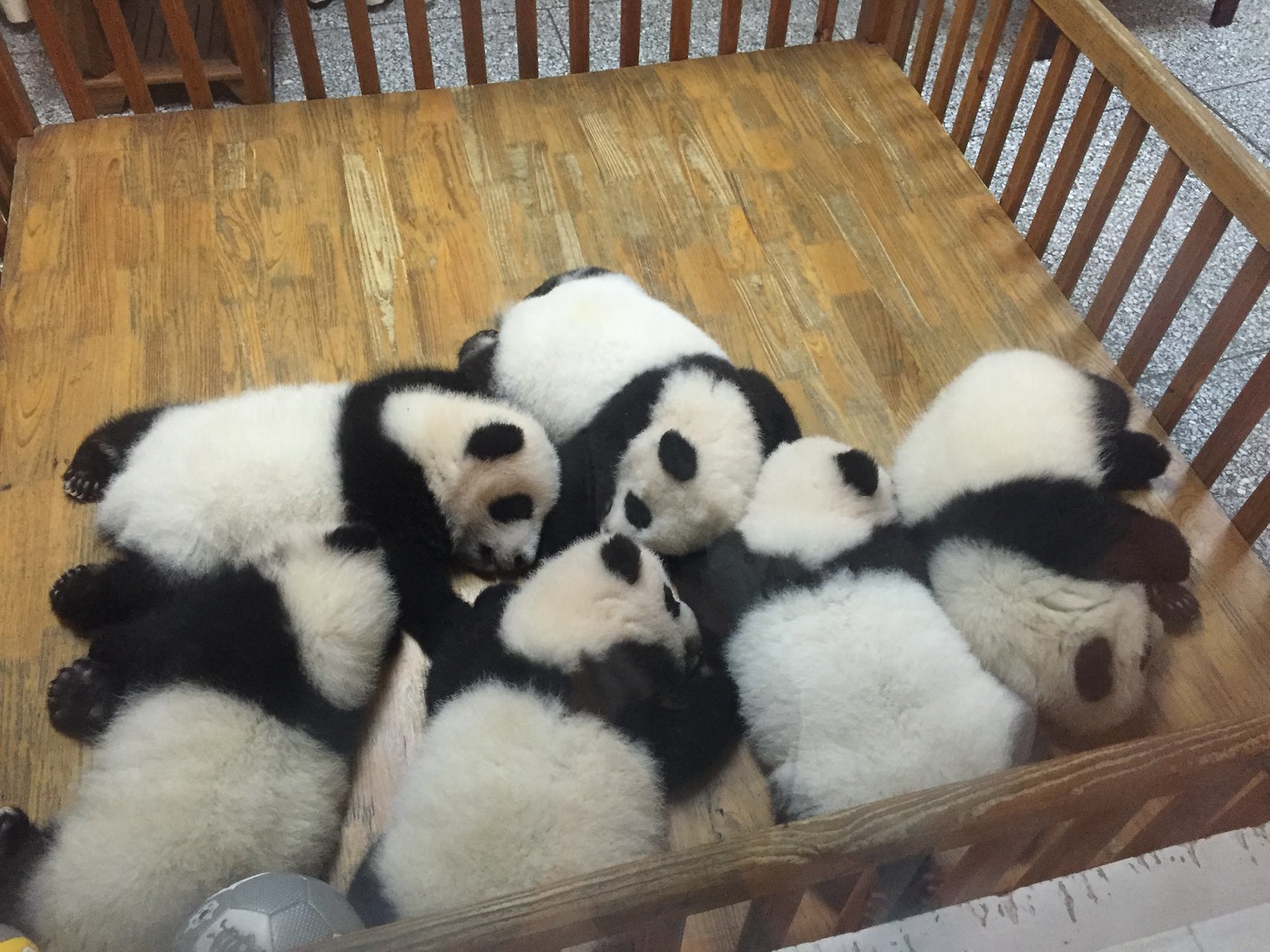In this detailed color photograph, a crib-like wooden pen is seen, made of a light brown, square-shaped wooden floor with vertical wooden bars forming a low railing around its perimeter. The wood of the railing is a slightly darker shade of brown, providing a sturdy barrier to prevent escape. Inside this pen, situated primarily towards the bottom right corner, lie six adorable baby panda bears, all in various sleeping positions. Their fur is predominantly white, contrasted with distinctive black patches around their eyes, black ears, black limbs, and a black band around the neck region. They rest peacefully, some sprawled on their stomachs while others recline on their sides. Among the slumbering cubs, a small gray ball, resembling a volleyball, adds a touch of playful charm. The background reveals a gray, tiled floor, but the focal point remains on the charming, tranquil scene of the snoozing panda cubs within their cozy wooden enclosure.